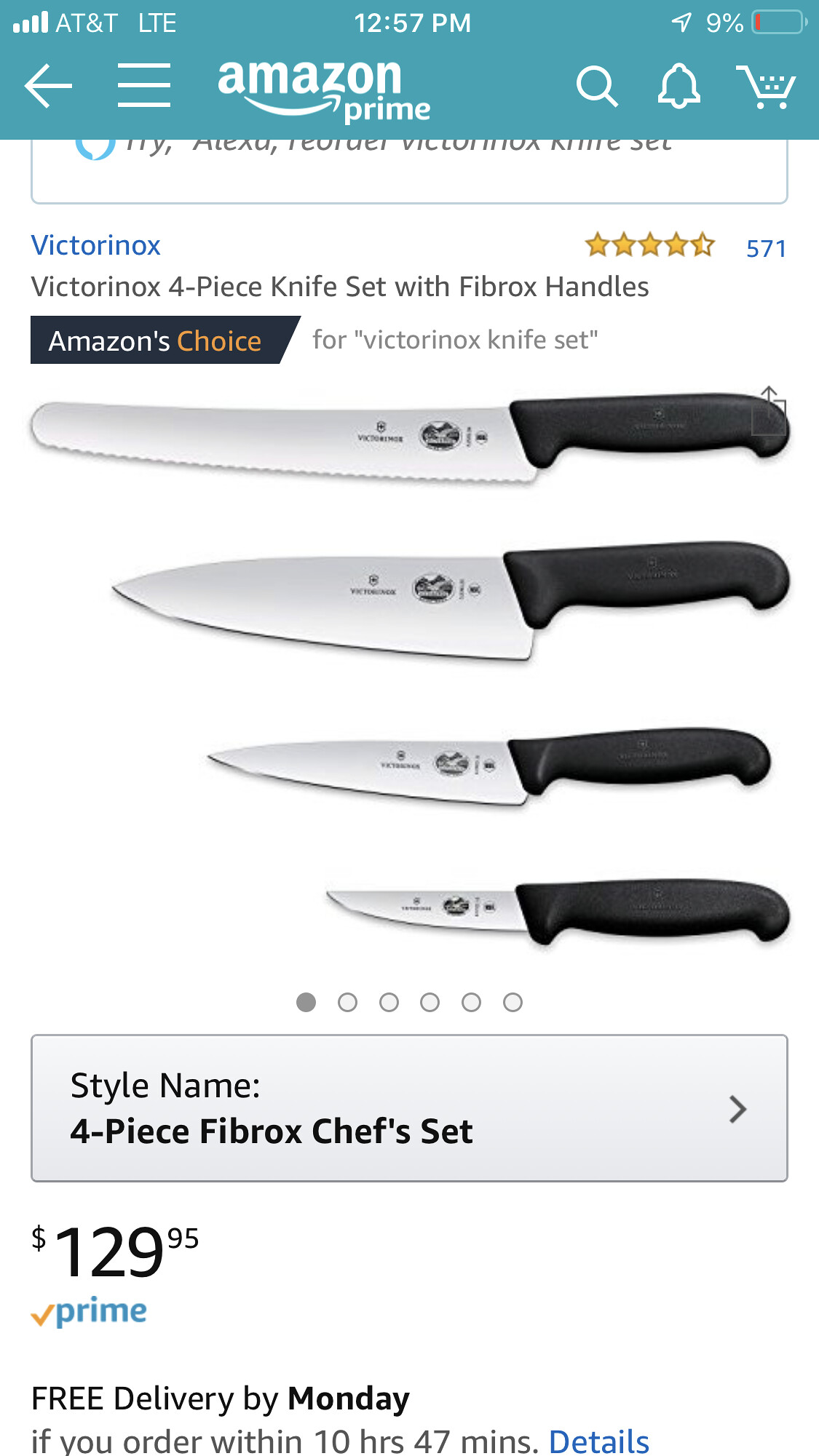This screenshot from an Amazon Prime listing showcases a Victorinox four-piece knife set with Fibrox handles, priced at $129.95. The knives, including a thin, long knife, a butcher's knife, a fillet knife, and a paring knife, all have black handles and silver blades. The listing indicates that it has a 4.5-star rating from 571 reviews and is labeled as Amazon's Choice. If ordered within 10 hours and 47 minutes, it promises free delivery by Monday. The screenshot, taken on a mobile phone using AT&T's LTE network at 12:57 p.m., shows the phone's battery at 9%. The top bar of the screenshot includes a back arrow, a menu icon, a search magnifying glass, a notification bell, and a shopping cart icon, all set against a light-blue background.